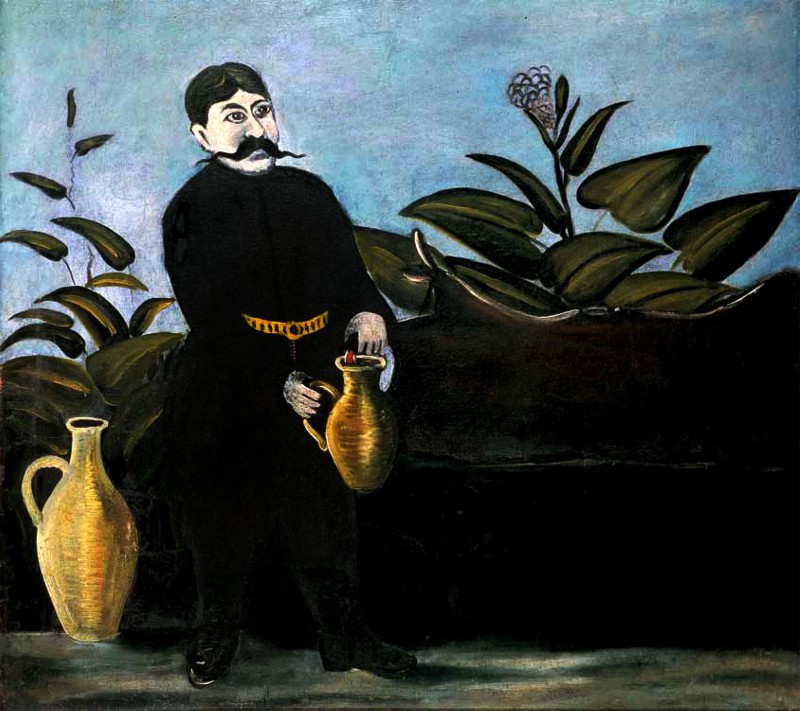The image depicts a painting of a solemn man with a distinguished long black mustache, black hair, and pale white skin. He is dressed in an elegant all-black jumpsuit with matching black shoes and is accented by a striking gold belt. The man, positioned on the left side of the image and facing forward, holds a golden vase with a handle in his right hand while standing amidst a lush garden setting. 

To his left, at the bottom of the image, there is a larger, lighter yellow-gold vase resting on the ground. Above this vase, some vibrant green plants add to the garden ambiance. On the opposite side, at the man's shoulder height, another plant with a delicate purple bud can be seen. The background of the painting features a mix of light blue and green hues, enhancing the serene yet contemplative atmosphere of the scene. The man appears deep in thought, perhaps even anxious, as he tends to the plants around him.